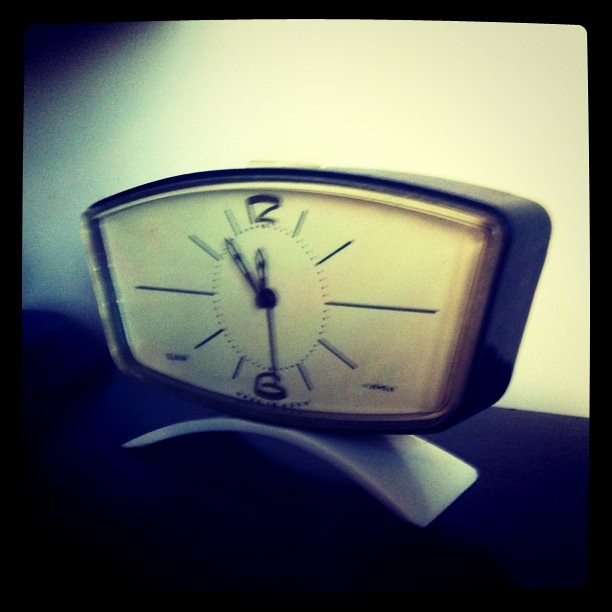This close-up image showcases a rectangular clock set against a divided background with black at the bottom and white at the top, possibly taken on a desk or table. The clock, which rests on a slightly tilted stand featuring a raised silver arch, dominates the central focus of the photo. Its outer frame is black with a clear plastic cover, encapsulating a white face adorned with minute markers represented as fine blue lines and small dots between them for the seconds. The clock prominently displays the numbers 12 at the top and 6 at the bottom, with three black hands in the center marking the time. The overall color palette includes shades of black, white, and gray, with the potential presence of navy blue. While there might be a brand name on the clock, it is not legible. The entire image is enclosed with a black border, enhancing its distinct, modern aesthetics.